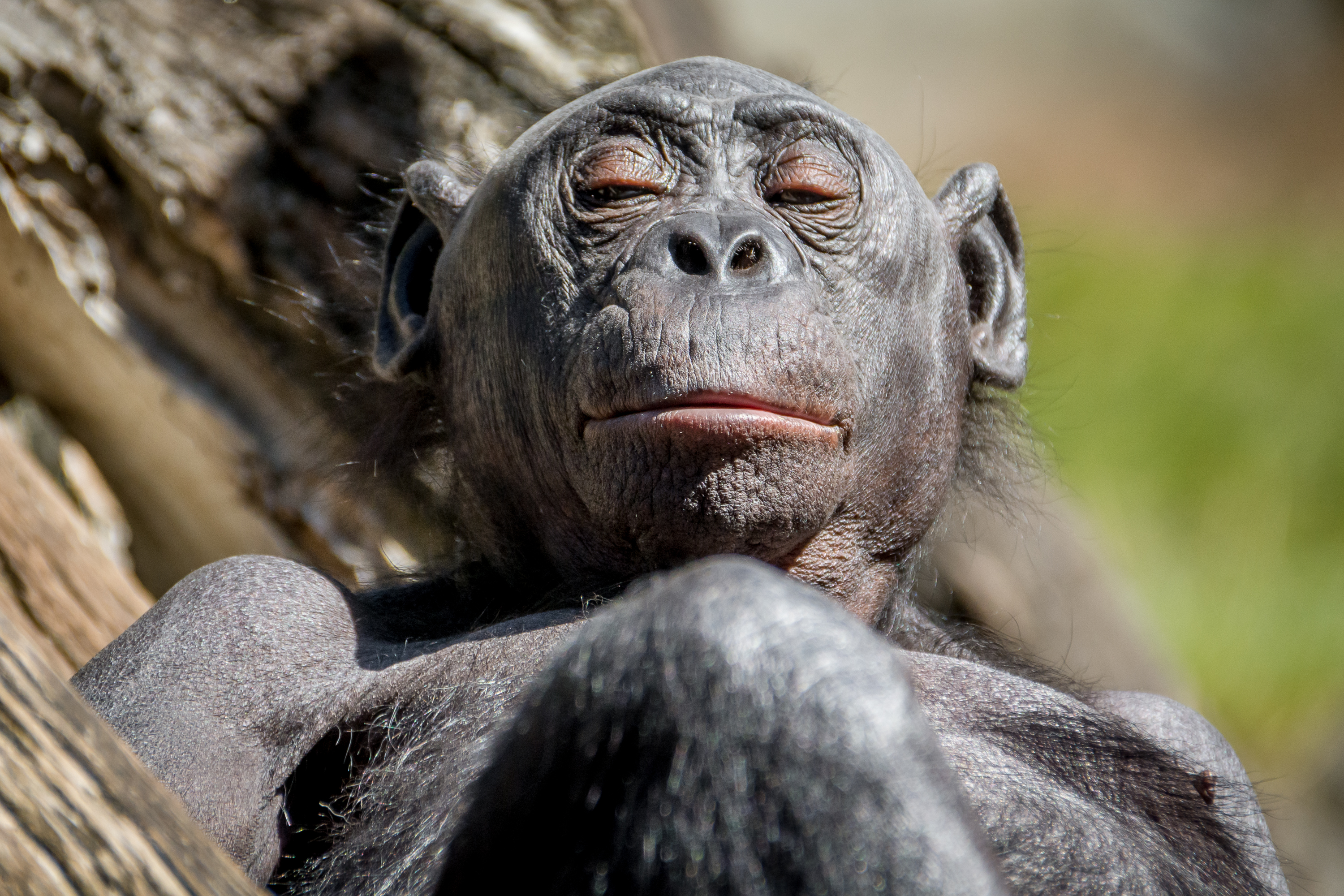This detailed photograph captures a reclining black monkey or chimpanzee. The animal, with its pink lips and eyelids, displays a bald head and patches of bald skin on its chest and legs, giving it an almost elderly appearance. Tufts of hair can be seen behind its ears. The monkey is resting on a sizable brown tree branch, with its eyes half-open, looking slightly annoyed or perhaps tired, as if disturbed from a nap. The background, blurred to bring focus on the animal, hints at greenery, possibly trees, bushes, or grass, suggesting an outdoor setting bathed in natural light.